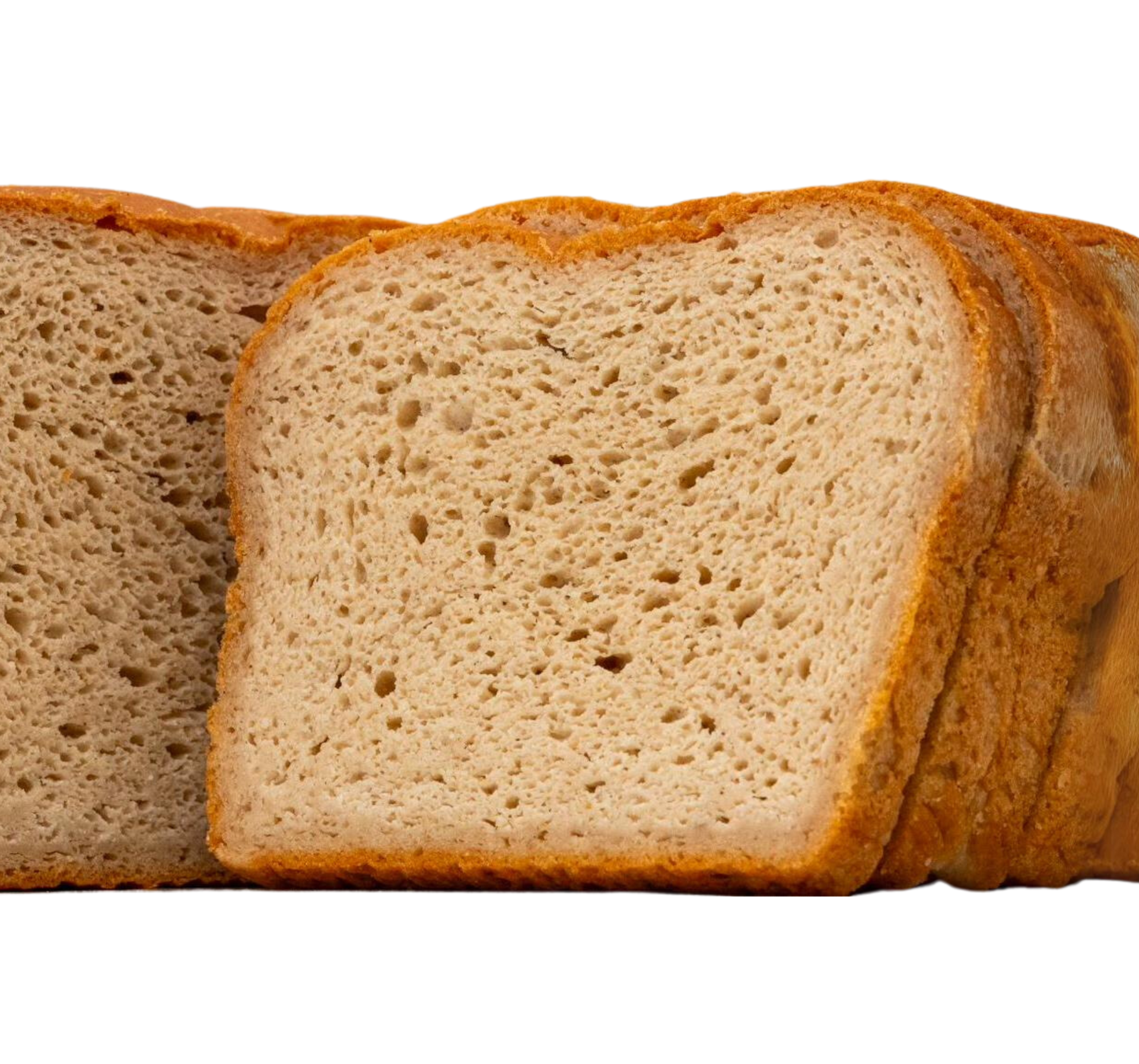This detailed close-up photograph showcases a freshly baked loaf of bread set against a white background. On the left side of the image, the whole loaf is visible, boasting a golden brown crust and a lighter beige interior indicative of its wheat or rye composition. To the right, the loaf has been sliced into five or six clean, thin pieces, each approximately half an inch thick. The bread's texture is porous, featuring varying sizes of holes—larger towards the center and diminishing towards the crust. The consistent golden brown crust and the distinctly softer, more porous middle suggest a freshly made bread that combines the characteristics of traditional white bread in its shape and size with the richer color and texture of wheat or rye.